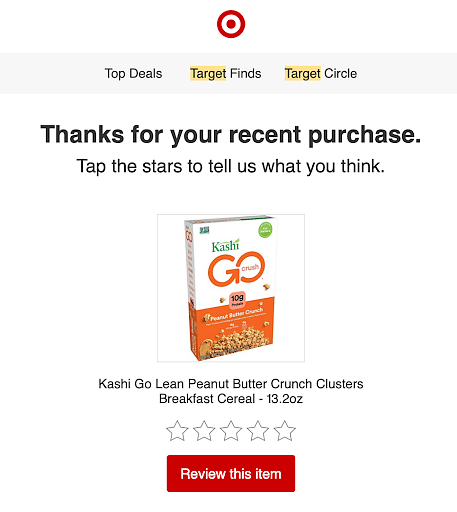This image showcases a feedback page from Target's website. The iconic Target logo, characterized by the red circle with the white inner circle and red dot, is prominently displayed. A gray bar stretches across the top, featuring sections titled "Top Deals," "Target Finds," and "Target Circle," with each section highlighted in yellow. Below this bar, a message expresses gratitude for a recent purchase and encourages the customer to "tap the stars to tell us what you think."

The customer had purchased Kashi GoLean Peanut Butter Crunch Clusters, a breakfast cereal available in a 13.2-ounce package. Beside the product name, an uncolored five-star rating system is visible, indicating that no reviews have been submitted yet.

Dominating the lower portion of the page is a large red box with white text that reads, "Review this item," urging the customer to provide feedback on their purchase. This feedback page is part of Target's post-purchase experience, aiming to gather customer reviews for future shoppers. The image ends here, focusing on the prompt for customer feedback.